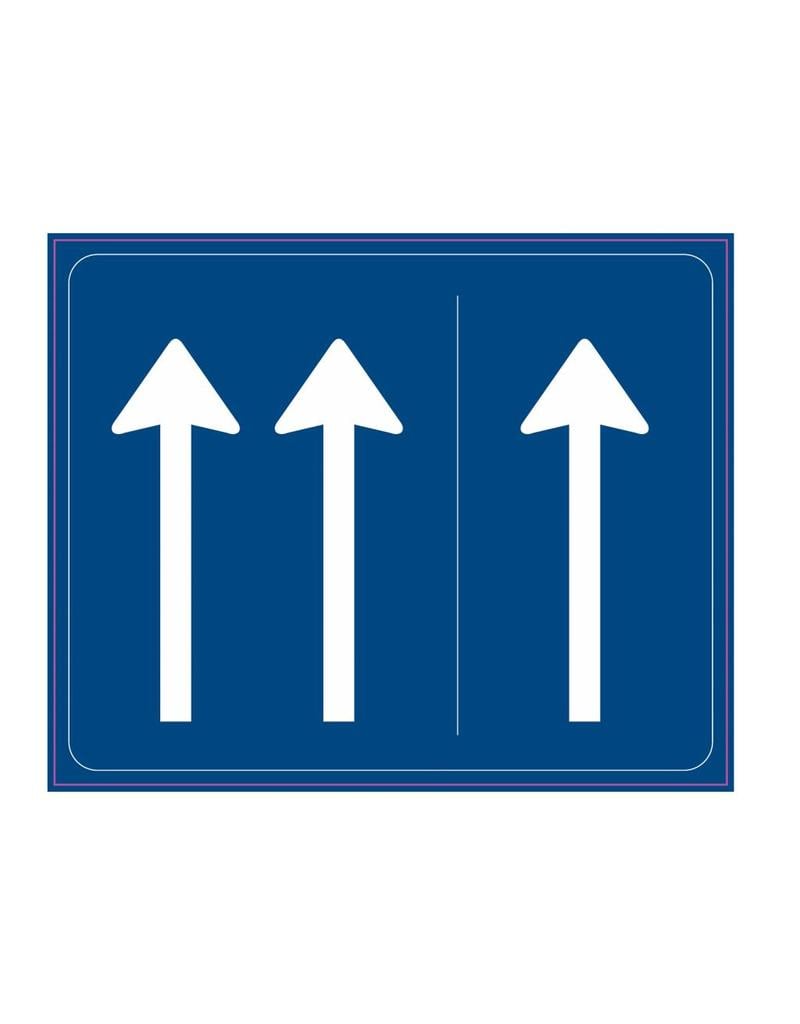The image is of a blue square traffic sign featuring a white rectangular border with rounded edges. Inside this border, there are three large, thick white arrows pointing upward. On the left side of the sign, two arrows are positioned next to each other, separated from a single arrow on the right side by a thin vertical white line. The arrows are of identical length, occupying most of the sign’s vertical space. The sign likely indicates that the two left lanes continue straight ahead, while the right lane may split off or diverge, suggesting different routes or directions for drivers.